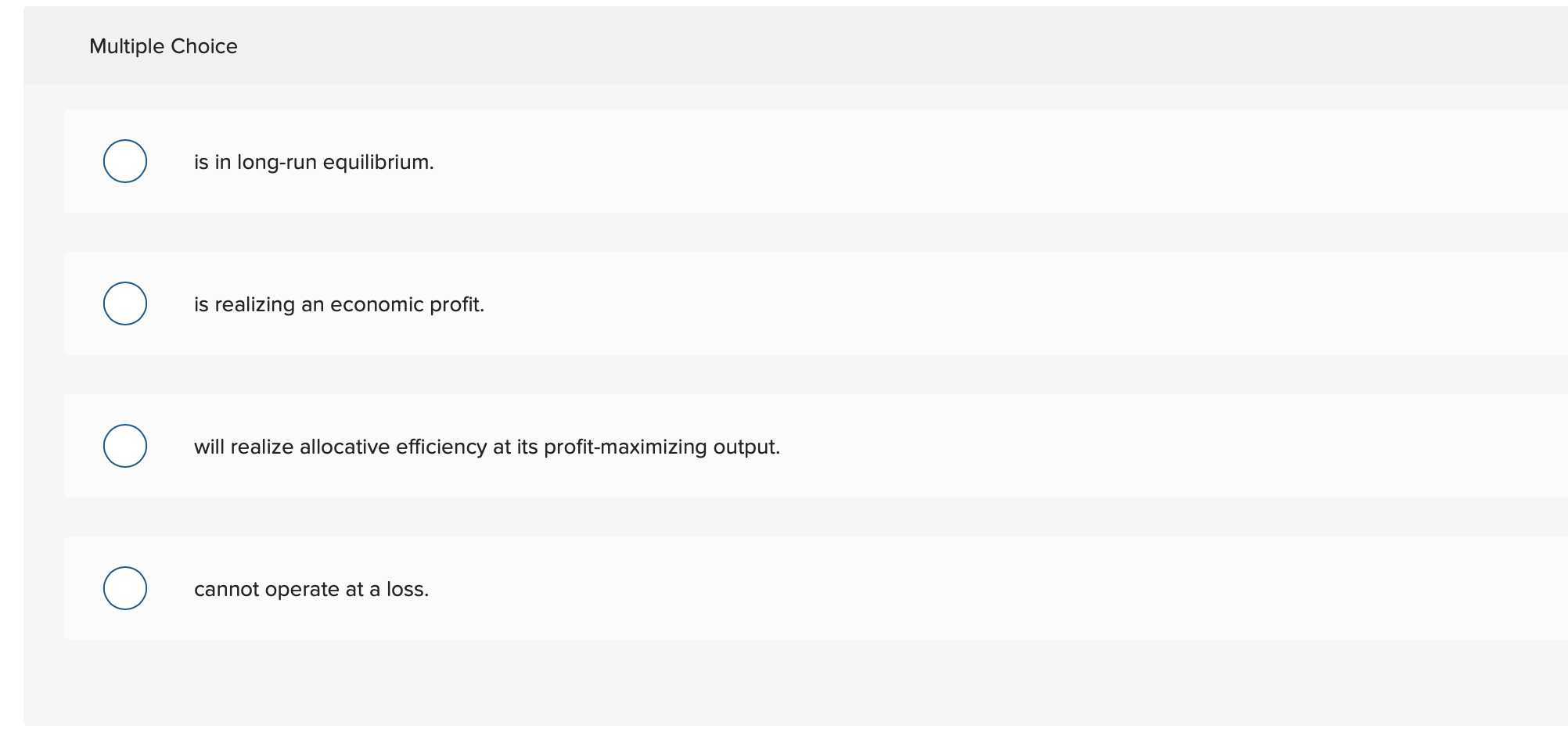**Detailed Caption:**

The image displays a rectangular area with a grayed-out background, divided into sections containing information. Situated at the very top within the grey border, the text "Multiple Choice" is prominently displayed. Below this heading, there are four statements, each housed in solid white blocks within the gray rectangle. Each block of text is spaced out with significant triple spacing between them.

1. The first block contains a round circle outlined in blue, followed by the text "In long-run equilibrium," written in small black print.
   
2. The second block, formatted similarly, includes a circle outlined in blue and the text "Realizing an economic profit."

3. The third statement, structured identically to the previous ones, features the blue-outlined circle, followed by "Will realize allocative efficiency at its profit-maximizing output."

4. Lastly, the fourth white block displays another circle outlined in blue, alongside the text "Cannot operate at a loss."

Each piece of information is meticulously organized and clearly delineated within their respective white blocks, making the distinctions among the multiple choices evident.